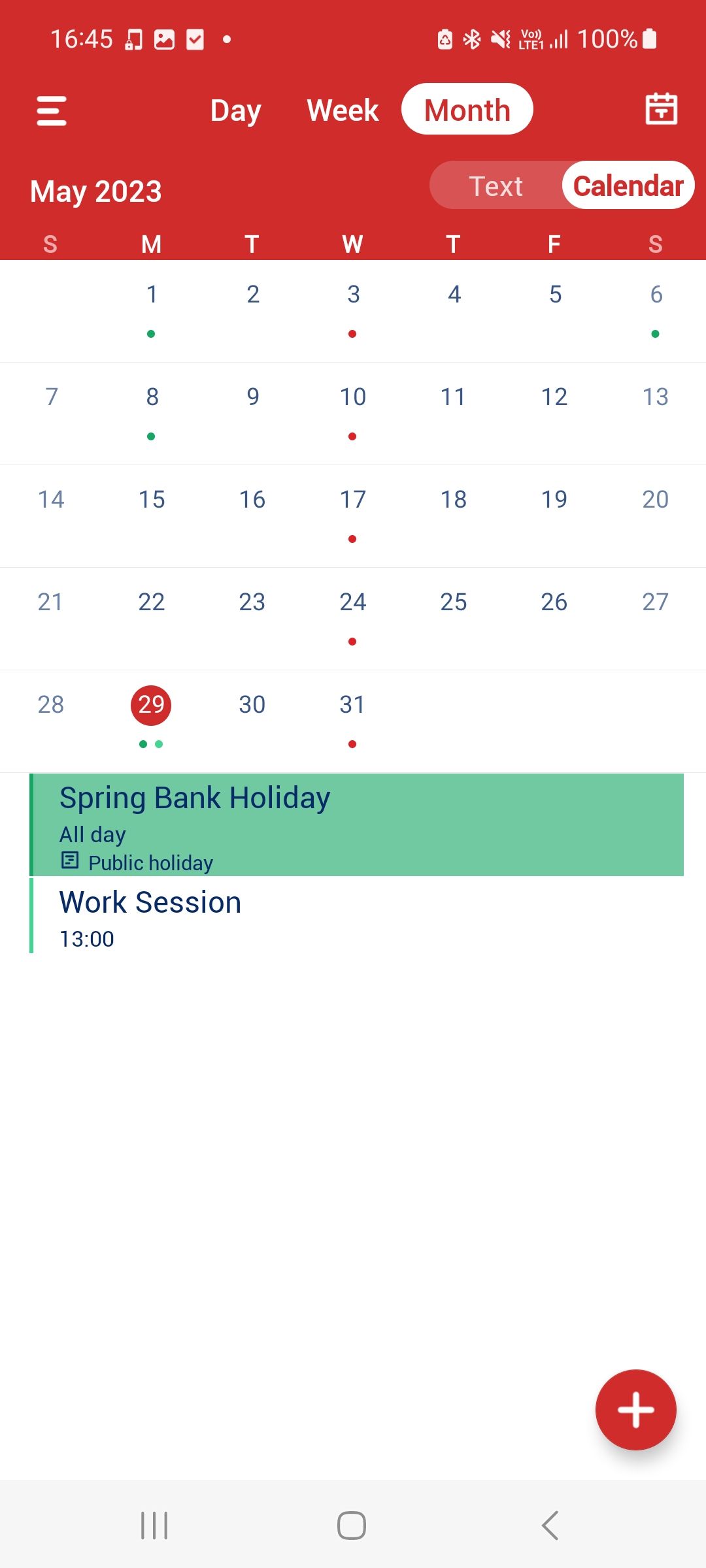This image is a detailed screenshot from a cell phone's display showing a calendar interface. The screen's top section features a vibrant red background displaying the time "16:45" in the top left corner and a fully charged battery icon at 100% on the opposite side. The primary section of the interface reveals an open calendar app, specifically focused on the "Month" view, indicated by a white circle around the "Month" tab—which sits amongst the "Day," "Week," and other options.

The calendar displays the layout for May 2023, starting with Monday the 1st and ending on Wednesday the 31st. Notably, May 29th is highlighted with a red circle, denoting it as a significant date. This date also features a blue background with the label "Spring Bank Holiday, Old Day, Public Holiday." Additionally, there is a scheduled work session at 13:00 on May 29th.

Towards the bottom right corner of the screen, there is a prominent red circle featuring a plus sign, suggesting that tapping it would allow the user to add a new event to the calendar. At the very bottom of the screen, a set of three horizontal gray lines flanked by a small circle are present, with a left-pointing arrow situated on the left side, indicating navigation options, possibly to return to a previous screen or menu.